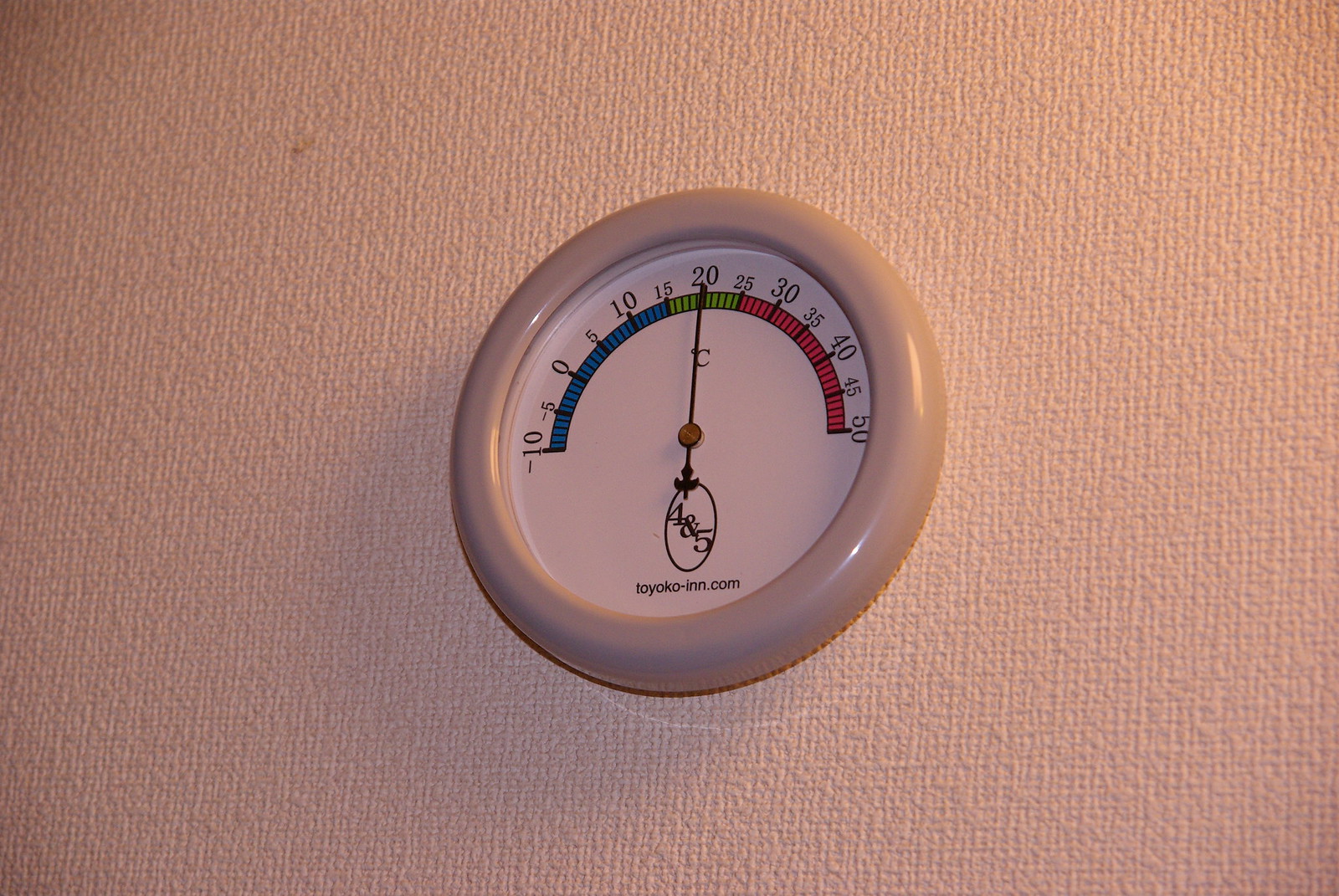The image depicts a white thermostat mounted on a textured, off-white wall. The wall appears slightly grainy and bumpy, giving it a gritty feel. The thermostat itself is primarily white, with an off-white frame that reflects some light. The display of the thermostat features a half-circle grid, ranging from -10 to 50 degrees. The temperature scale is color-coded: blue for -10 to 15 degrees, green for 15 to 25 degrees, and red for 25 to 50 degrees. The hand of the thermostat is precisely pointing at 50 degrees. Beneath the hand, within an oval, are the numbers "4" and "5," followed by the text "tokyo-in.com," suggesting that this thermostat is located at a hotel or inn in Tokyo.